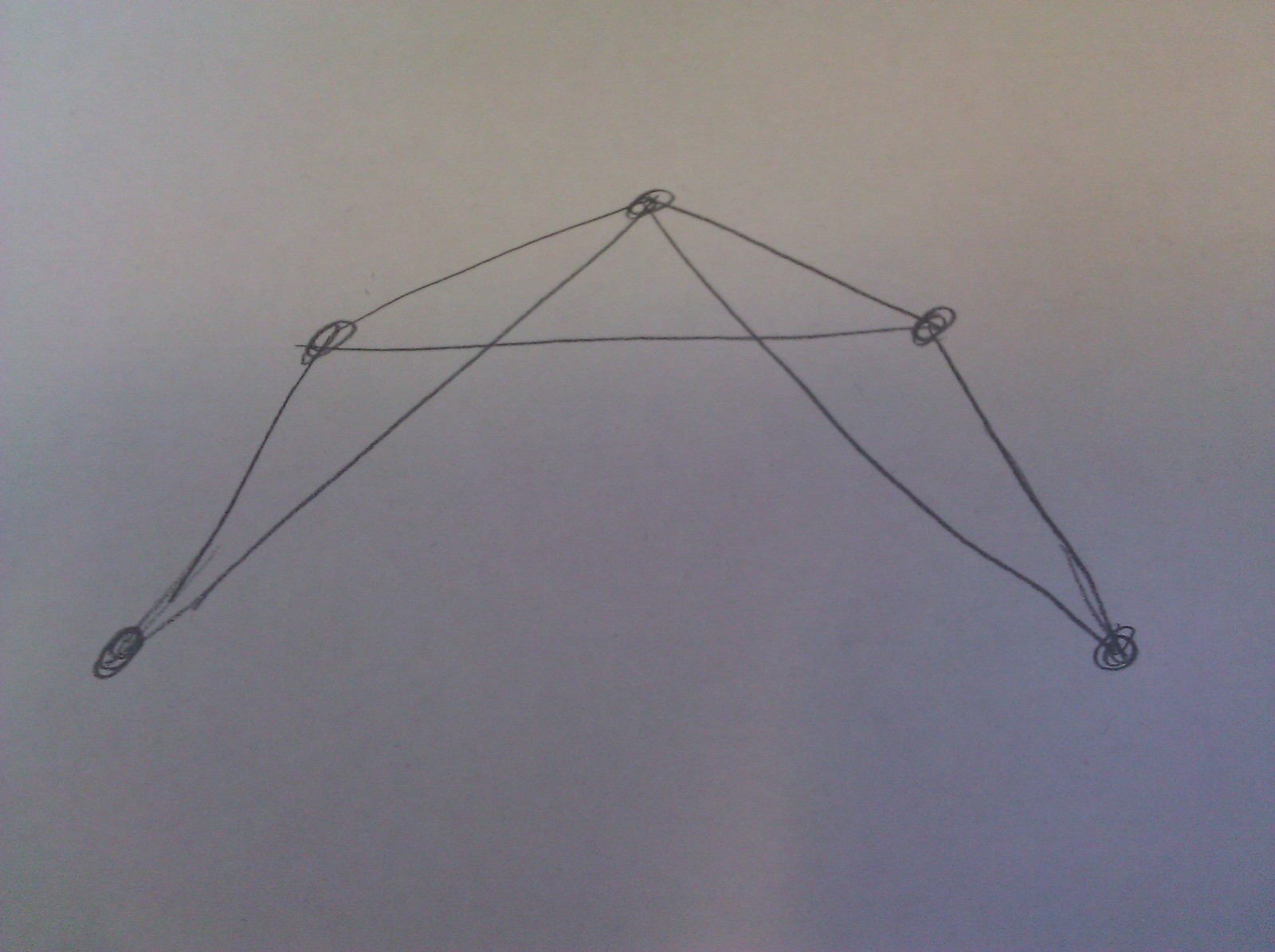The photograph captures a simple geometric line drawing on a white sheet of paper, presented in a horizontally aligned rectangle. The white paper appears slightly grayed due to subtle shadowing, which transitions in a smooth gradient from a darker shade in the lower two-thirds to a lighter shade in the upper one-third.

The drawing itself is rendered in a dark gray pencil, almost black, and features an abstract, stylized 'A' shape. This 'A' is composed of thicker, gently curved lines. Five circles filled with scribbles are scattered where the lines intersect, except at the central crossing of the 'A'.

The 'A' incorporates an extended horizontal line that exceeds the width of the letter. At each end of this horizontal line, a scribbled circle is drawn, with lines connecting from these circles down to the outer tips of the 'A', creating a pyramid-like form. The lines themselves are not perfectly straight but have slight curves and occasional corrections where the artist deviated from the intended path and doubled back without erasing the original marks. The overall effect is a blend of geometric precision and organic imperfection.